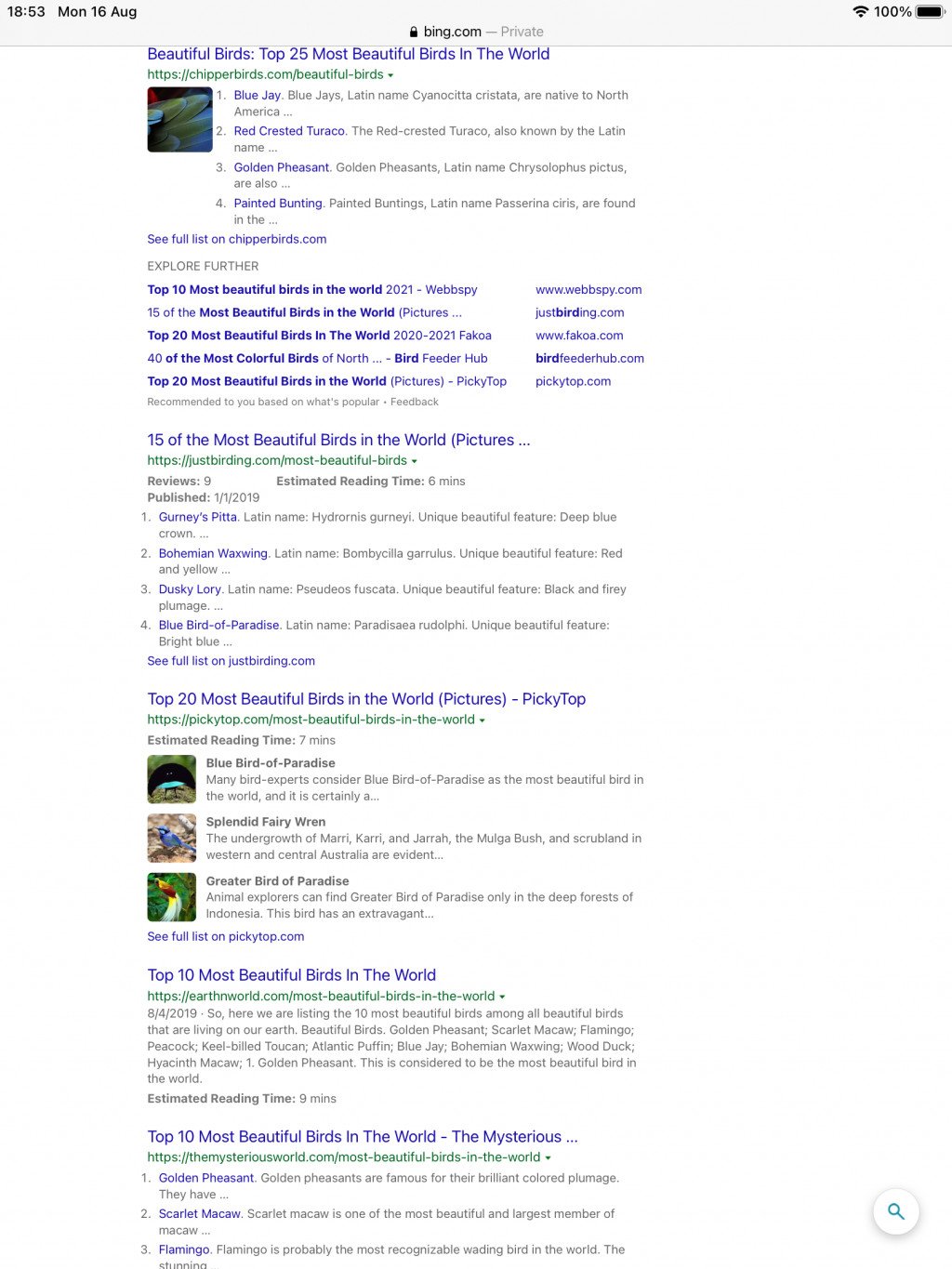The image displays a smartphone screen with a predominantly gray theme. At the top, there's a gray border displaying various status indicators. The current time is shown in black as "18:53," followed by the day "MON" for Monday and the date "16 AUG" for August 16th. Appearing centrally in black text is "bing.com," with a gray dash and the word "private."

To the right on the status bar, black icons indicate a full Wi-Fi signal, 100% battery, and additional connectivity features.

Below, in blue text, a headline reads, "Beautiful Birds: Top 25 Most Beautiful Birds in the World." A list of birds mentioned in the text includes the Blue Jay, Red-crested Turaco, Golden Pheasant, and Painted Bunting, with a prompt to see the full list on chipperbirds.com. Additional captions in gray and blue detail more lists and resources related to beautiful birds, including:

- "Top 10 Most Beautiful Birds in the World 2021" (websi)
- "15 of the Most Beautiful Birds in the World" (pictures)
- "Top 20 Most Beautiful Birds in the World 2021" (flaco.com)
- "40 of the Most Beautiful Birds of North America" (birdfeederhub.com)
- "20 Top Most Beautiful Birds in the World" (pickytop.com)

Other sections include references to articles such as "Top Most Beautiful Birds in the World" (earthworld.com) and "The Mystery World: Top Most Beautiful Birds" (themysteryworld.com). Each resource provides additional context and visual content concerning the most beautiful bird species globally.